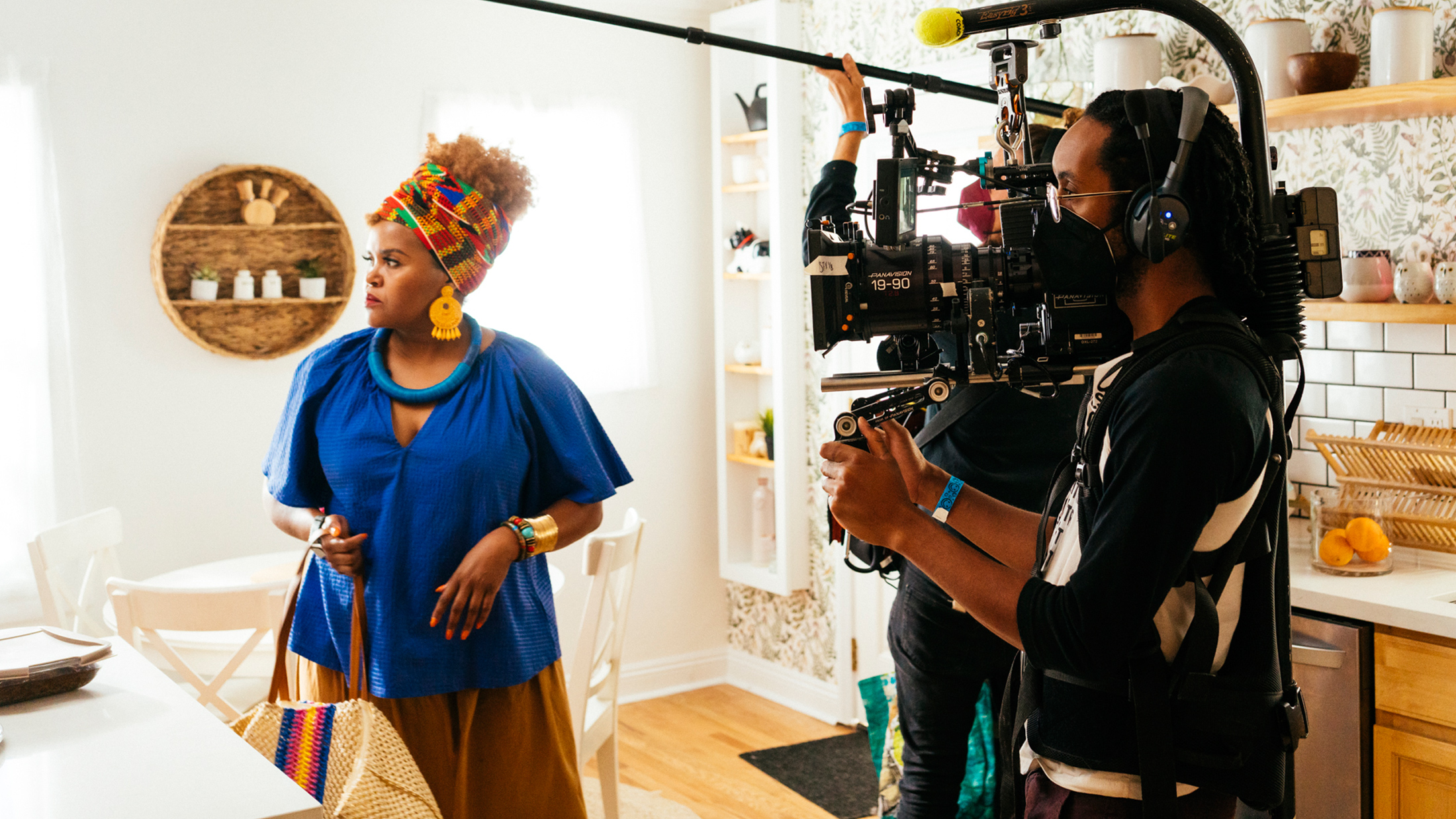In this vibrant color photograph, a film crew is capturing a scene in a home kitchen. On the left side of the image, a dark-skinned woman, likely African-American, stands out. She is wearing a flowing, blue tunic-style top and a brown skirt. Her hair is adorned with a multicolored headdress featuring hues of orange, brown, green, blue, and red, complemented by large yellow earrings. In addition, she sports a blue ring-like necklace. She is positioned in front of a white wall, with a white table in the foreground and another white table with chairs in the background.

On the right side, a male cameraman, also with dark skin, is engrossed in filming. Dressed in a black top with white accents and wearing a blue bracelet on his wrist, he handles a large video camera, which is supported by a comprehensive setup. Beside him, another crew member holds up a filter. The kitchen background also features white walls, a white backsplash, a counter, a stainless steel refrigerator, and shelves holding plants and a glass bowl filled with oranges. This detailed setup captures the essence of the scene being filmed, highlighting both the characters and their environment vividly.